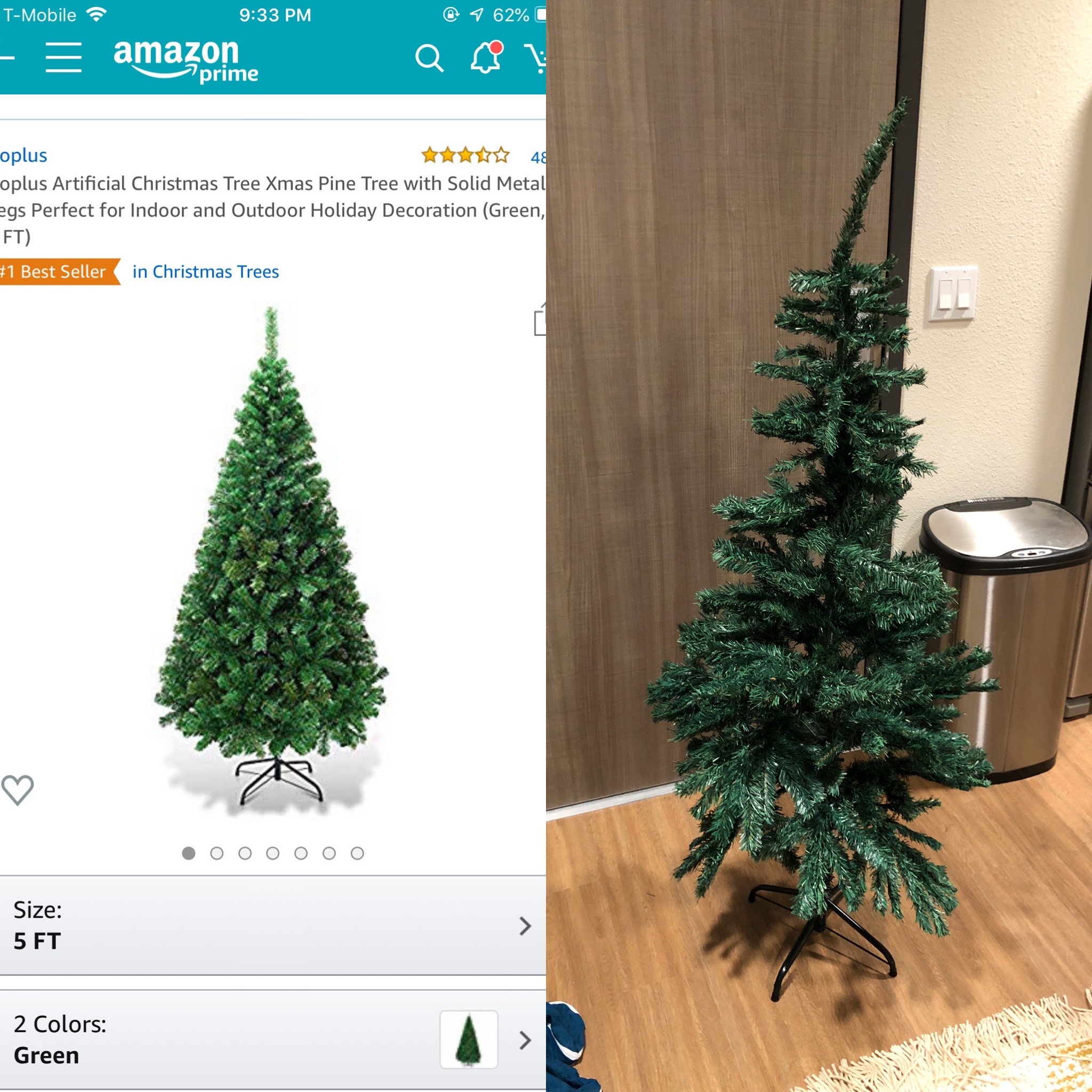The image showcases a scene at 9:33 PM, where a T-Mobile device is connected to Wi-Fi. A detailed view of a kitchen reveals it is over 60% occupied. There is a hint of Amazon Prime subscription usage. Notably, there are icons including a UNDC logo, a magnifying glass, and a bell with a red dot, indicating notifications. 

Prominently featured in the image is an artificial Christmas tree, marketed as an "Opalist," adorned with three and a half gold stars. The tree is described as a Christmas pine tree with solid metal construction, making it ideal for both indoor and outdoor holiday decorations. The tree holds the title of the number one bestseller in Christmas trees on Orange. The structural base includes metal legs. A dark grey element, resembling half a heart, is visible along with six hollow circles.

A grey bar indicating the size of the tree, "5 feet," and its colors being green, is present. To the right of the tree stands a brown wooden door. The setting includes a wall with light switches and a trash can nearby. The Christmas tree is dusted with artificial snow, enhancing its festive appeal. Below the tree is a rug with visible strands, and in the bottom left corner lies a blanket on the floor. The door and floor are accented with greenery, and there is a shadow casting over the area.